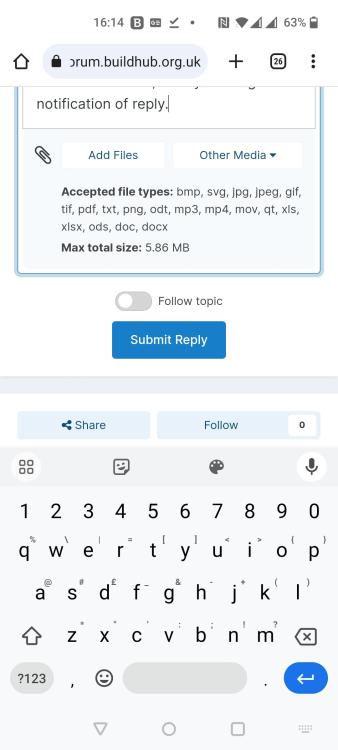In the image, we observe a smartphone screen displaying a notification on an app, likely a forum platform, specifically buildhub.org.uk. At the top of the screen, the phone's status bar is clearly visible. The main content of the screen shows a notification titled "Notification of Reply," indicating that the user has received a response to a previous post or comment. Below this notification, there is a section titled "Add Files or Other Media," which provides a list of accepted file types for upload, including BMP, SVG, JPEG (listed twice with slightly different formatting), GIF, TIFF, PDF, text, PNG, ODT, MP3, MP4, MOV, QT, XLS, ODS, DOC, and DOCX, with a maximum total upload size of 5.86 megabytes. Further down, there is a "Submit Reply" button, and at the bottom of the screen, an on-screen keyboard is visible, ready for the user to type out their message.